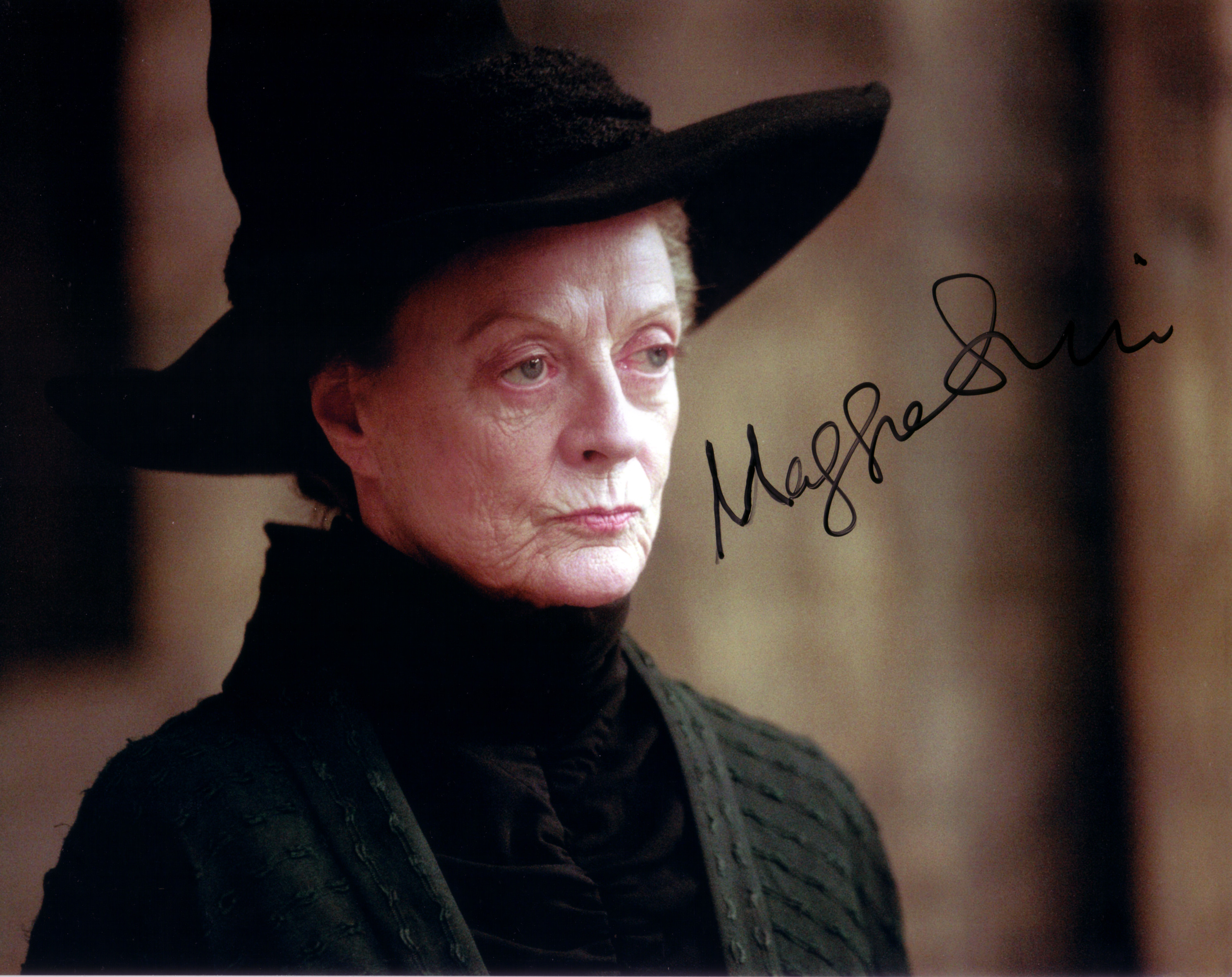The image portrays a distinguished actress, seemingly in her late seventies, known for her role in the Harry Potter series. The photograph, likely a still from the movie, features her in character, donning a traditional black witch's hat. The hat boasts a wide brim that casts a shadow over her face and has a pronounced pointed peak in the center. She exudes a calm and composed demeanor, her gaze directed off-camera, adding an air of mystery and introspection to the scene.

The actress is clad in a dark, intricately detailed outfit. The garment resembles a turtleneck suit, its fabric textured with visible ridges that add depth to the ensemble. The top part drapes elegantly over her chest, and an additional dark undershirt peeks from beneath. To the right of her serene visage, her autograph is gracefully inscribed in a black cursive script, lending a personal and cherished touch to the photograph.